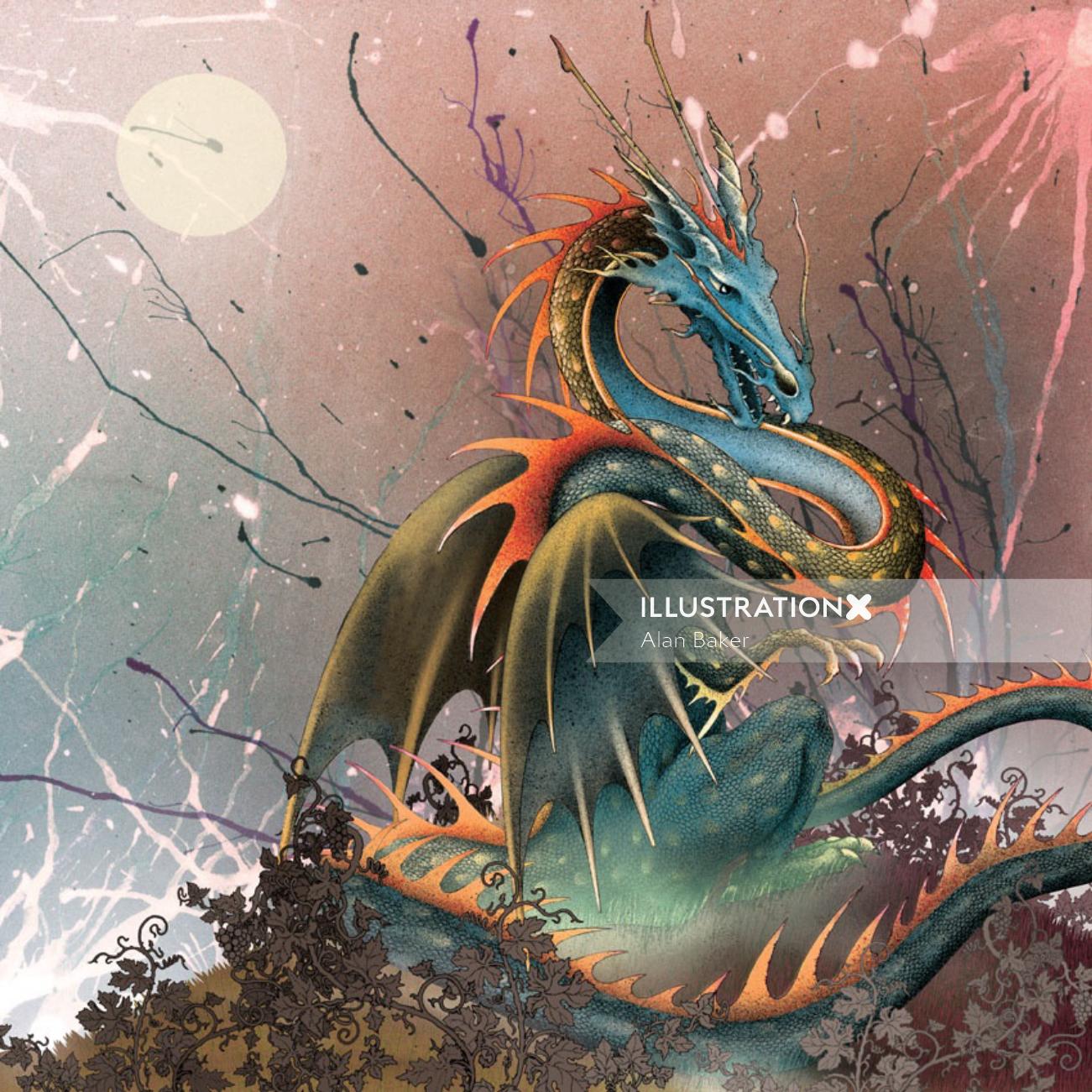The image is a detailed digital illustration of a dragon inspired by traditional Chinese art, centered in a background that transitions from light blue on the left to pink and purple on the right. The dragon's body is intricately curved, featuring a striking blue head with two root-like structures extending from its nostrils, and fierce black eyes. Its elongated head faces to the right and sports short, pointed ears with thin, horn-like antlers atop. The neck, adorned with goldish spots and a blue underbelly, leads into a green-scaled body with dark yellow patterns, resembling a serpentine blend of a slug and a prehistoric creature.

The dragon's hind legs bear a resemblance to a dinosaur's, and its forelimbs are short, stocky, and clawed, with orange spiked tendrils on the elbows. Two large green wings extend from its back, contributing to its majestic presence. Its long, winding tail, edged with orange fin-like spikes, circles around the dragon, creating a dynamic sense of movement. 

The scene is enriched by the addition of leaves and flowers interwoven among the dragon's limbs and back, painted in greenish-yellow tones. The background includes splashes of dark blue, purple, and black, adding an element of dramatic action. A perfectly round, cream-colored circle in the upper left corner suggests a celestial body, contributing to the mystical atmosphere. The illustration, attributed to Alan Baker, is both professional and captivating, capturing the essence of a mythical, regal dragon set against a vibrant, action-filled backdrop.